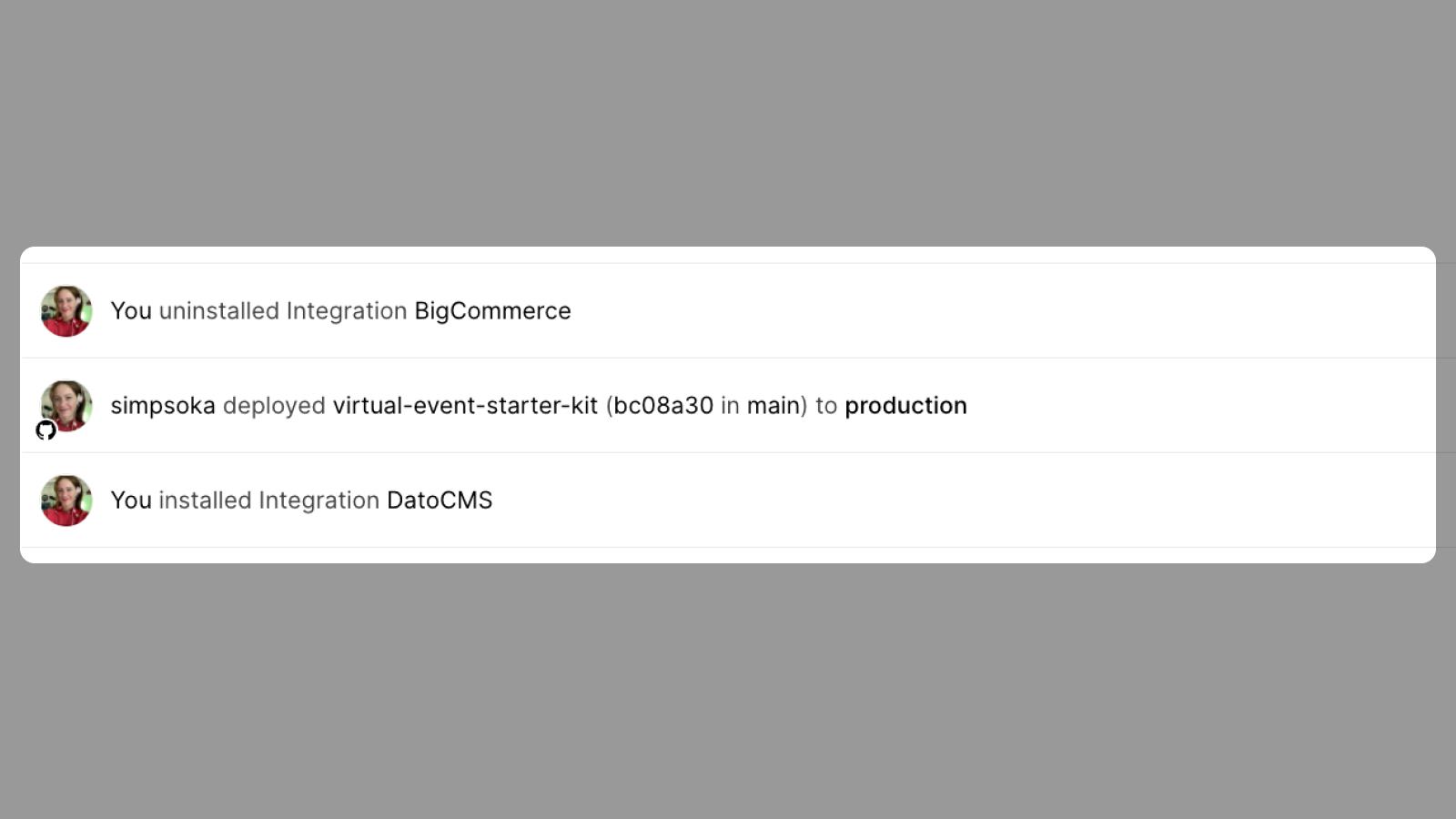The image features a gray rectangular background with a white, centrally placed rectangular shape that has rounded corners. Inside, the white rectangle is divided into three distinct sections by four gray lines. 

In the first section, on the left side, there is an icon displaying a woman with long brown hair wearing a red shirt. Next to this icon, bold text indicates: "You uninstalled integration BigCommerce," with "You" and "BigCommerce" emphasized.

The second section displays a GitHub icon in the bottom left corner. Adjacent to this, there is a closer view of the same woman's icon. The bold text reads: "Simp Soca," followed by gray text, "deployed," and then bold text: "virtual-event-starterkit (bc08a30) in main to production."

In the third and final section, similar icons are shown with the woman’s image again. The bold text states: "You installed integration .o cms," with "You" and ".o cms" both in bold. The repeated icon sizes and placements emphasize the sequential actions taken.

The layout provides a clear, detailed series of events regarding installation and deployment activities, using varying icon sizes and bold text for emphasis.